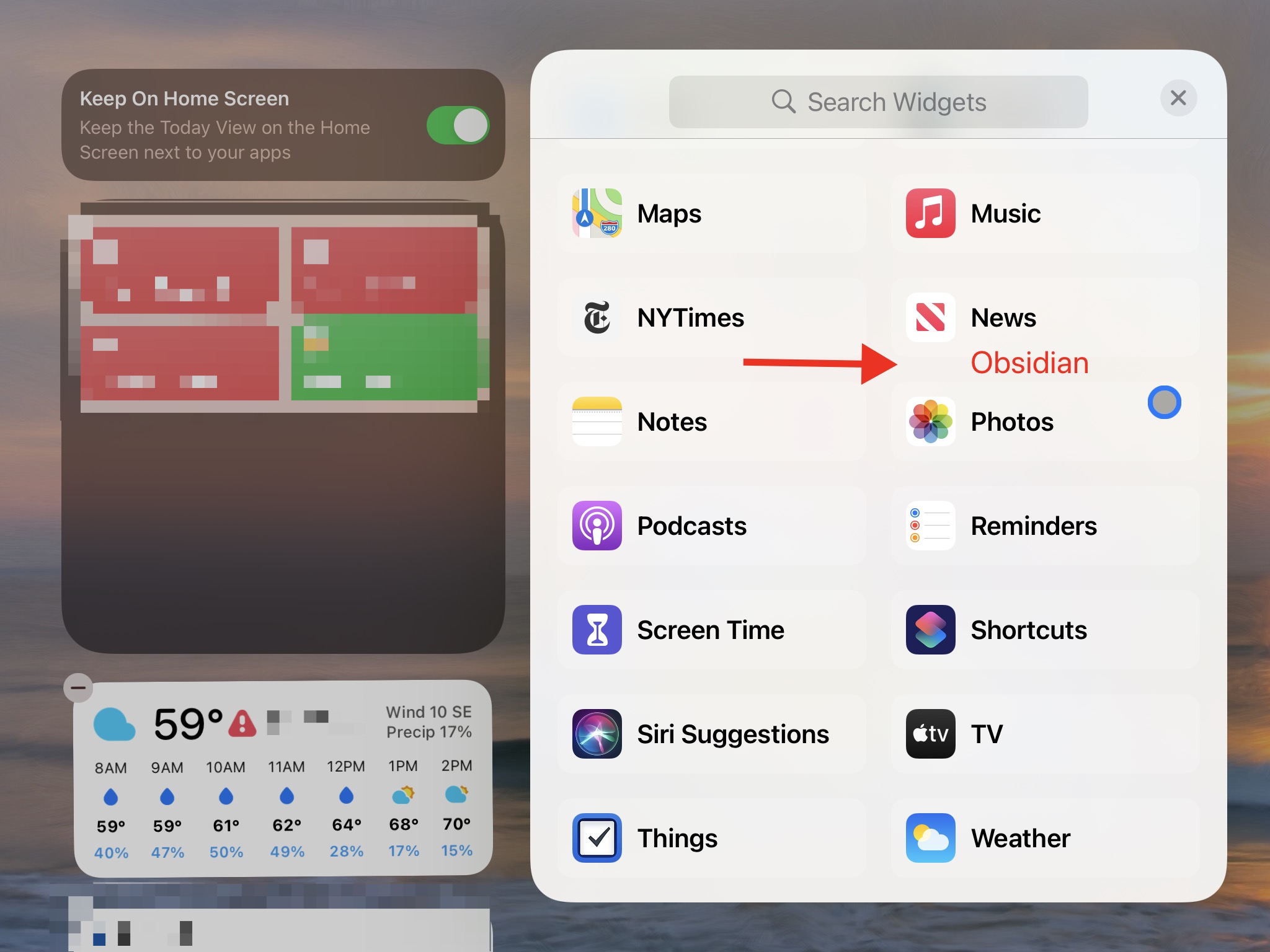This digital image features a detailed layout of a smartphone home screen. In the top left corner, the words "Keep on Home Screen" are displayed, suggesting an option to retain the Today View alongside the apps on the home screen. Directly beneath this, there's a weather widget indicating a temperature of 59 degrees Fahrenheit, with a southeast wind blowing at 10 mph and a 17% chance of precipitation. The temperature forecast for the morning and early afternoon is also detailed:

- 8 a.m.: 59°F
- 9 a.m.: 59°F
- 10 a.m.: 61°F
- 11 a.m.: 62°F
- 12 p.m.: 64°F
- 1 p.m.: 68°F
- 2 p.m.: 70°F

Several app icons are arranged below and around the weather widget, including Maps, The New York Times app, Notes, Podcasts, Screen Time (represented by a white hourglass), Siri Suggestions, Things, Music, News, Obsidian, Photos, Reminders, Shortcuts, Apple TV, and another Weather widget.